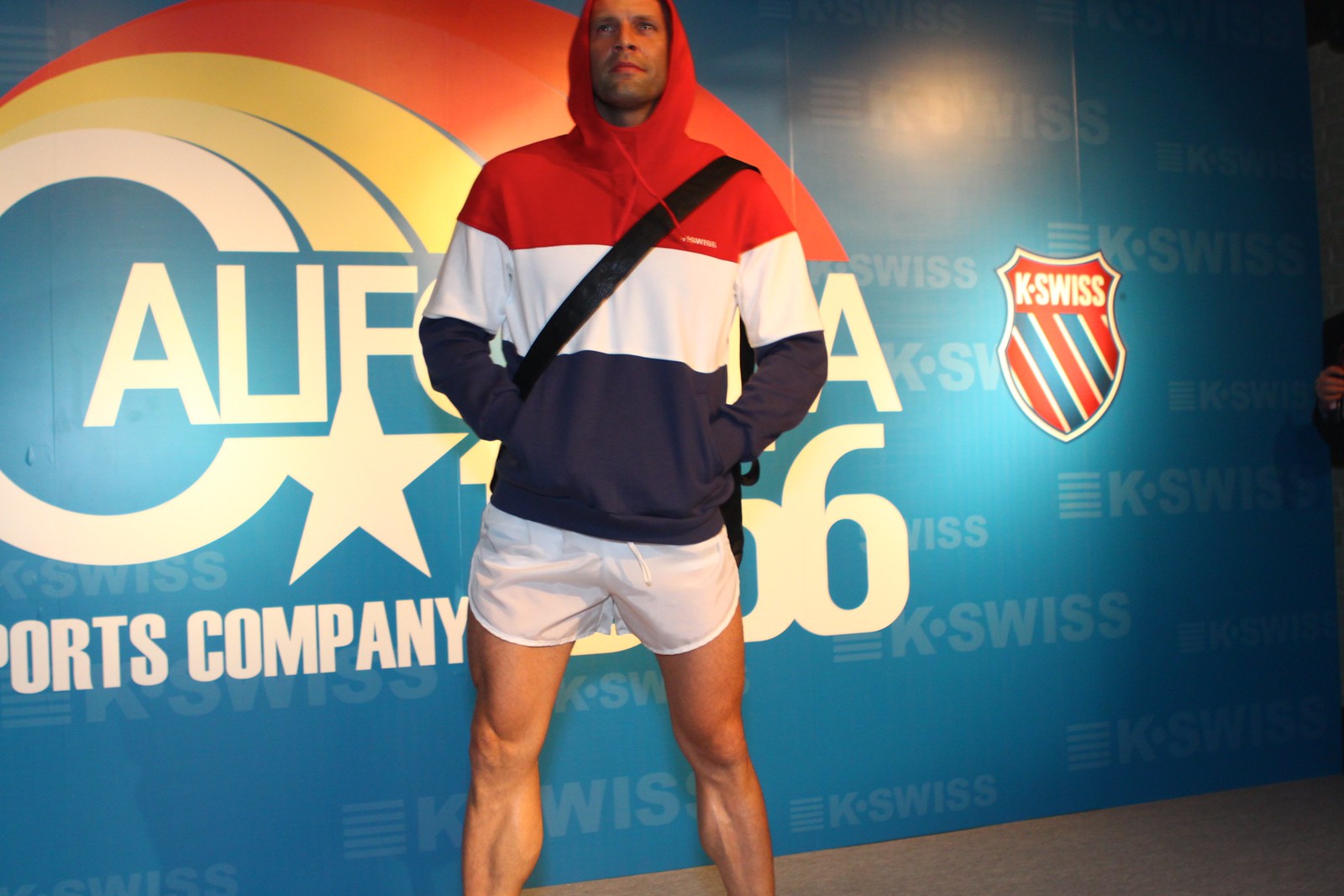A tall, muscular man stands confidently in front of an advertisement wall, partially obscuring its text and images. He wears a hoodie with a red top, a white central strip, and a blue bottom section, reminiscent of an American flag. The hood is up, covering his head and shoulders, and his hands are tucked into the hoodie's pockets. His lower half sports short white shorts, revealing his well-defined legs. A black strap from a bag runs diagonally across his chest, with the bag slung over his back. Behind him, the advertisement features a predominantly white background with ghosted K-Swiss logos and a distinct badge emblem with red and blue stripes. The visible text reads "sports company" and displays a partial word "C-A-U-F", which transitions into a rainbow design arching across the ad. The number 66 is also visible. Despite the partial obscuring by his tall frame, the context suggests this is a promotional event involving K-Swiss and athletic apparel.